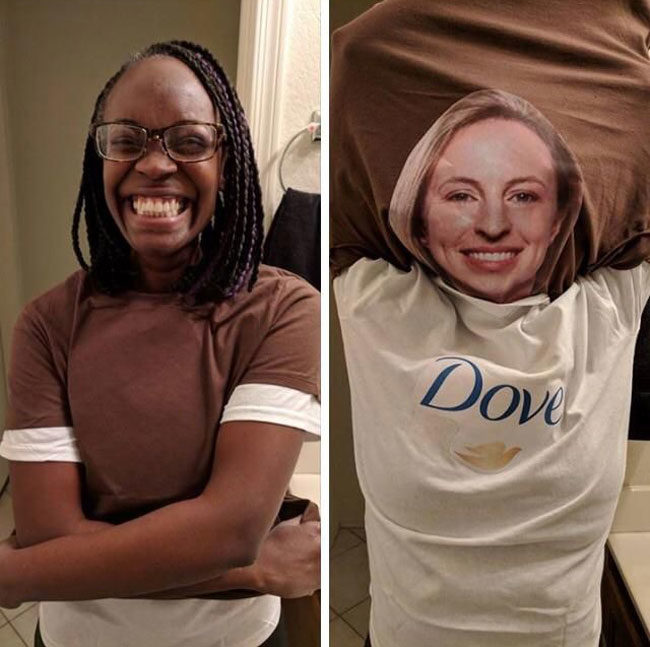The image is a vertically-aligned composite featuring two adjacent photographs. On the left, an African-American woman with shoulder-length braided hair and eyeglasses is smiling broadly with her teeth showing. She wears a short-sleeve brown shirt over a white t-shirt, with the bottom hem of the white t-shirt visible. Her arms are crossed, left arm over right, against a background consisting of a brown wall and a white window trim in the upper right corner. The right photograph showcases a cutout of a Caucasian woman's face, smiling with lipstick on, placed over a white t-shirt displaying the Dove logo in navy blue letters with a gold bird symbol beneath it. This cutout face appears superimposed and is not of an actual person. The background here is formed by a brown sheet draped across the wall, creating a humorous juxtaposition.